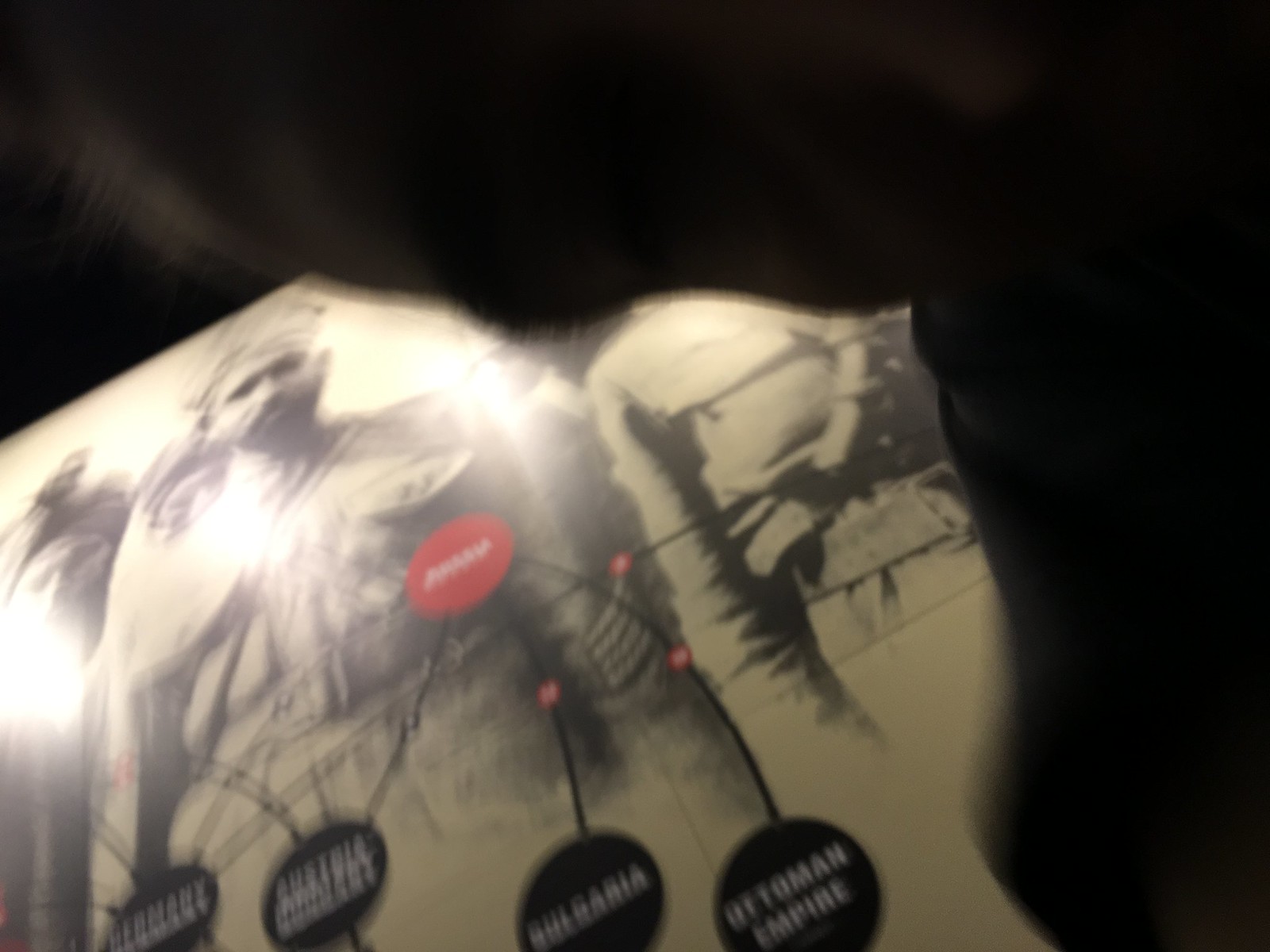The image is a blurry, partial photograph set against a black background, resembling a torn or ripped page from an old album. It depicts three military men dressed in uniforms, one of whom is fully visible in the center with a beard and hat and possibly wearing a turban, giving him a Middle Eastern appearance. The other two figures are less discernible; one shows only a torso on the right, while the third appears just behind the central figure, also possibly wearing a turban. The photo includes several labeled circles, displaying the names "Germany," "Austria," "Bulgaria," and "Ottoman Empire," hinting at a historical military context. Despite the lack of context and the presence of glare, it's clear that someone is looking at this image on a screen, perhaps confusing it as an advertisement or part of a game or movie due to its indistinct nature. The mixture of black and white elements, along with a single red and white label, adds to the aged and enigmatic feel of the photograph.